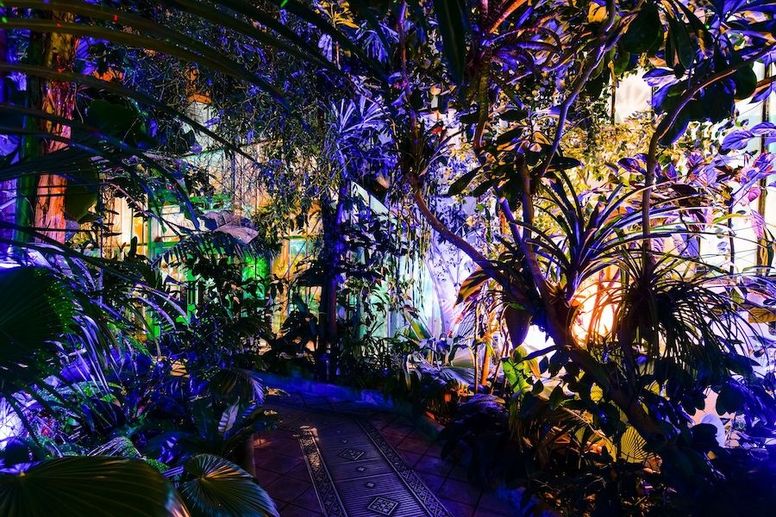This detailed, angled view of an indoor jungle reveals a dense, lush landscape adorned with a spectrum of colorful lights. To the left, blue lights cast a neon glow on the plants, while to the right, the foliage is bathed in hues of yellow, green, and purple. The garden is bisected by a distinct metal walkway featuring unique symbols, including diamonds and dots, curving gently to the left. Above, stained glass panels in the top left corner filter sunlight into a dazzling array of colors, illuminating the leaves and contributing to a mesmerizing, multi-hued effect. Large trees and branches arch over the scene, creating an intricate canopy that adds to the jungle's depth and complexity, while the peering light through the stained glass enhances the enchanting atmosphere.